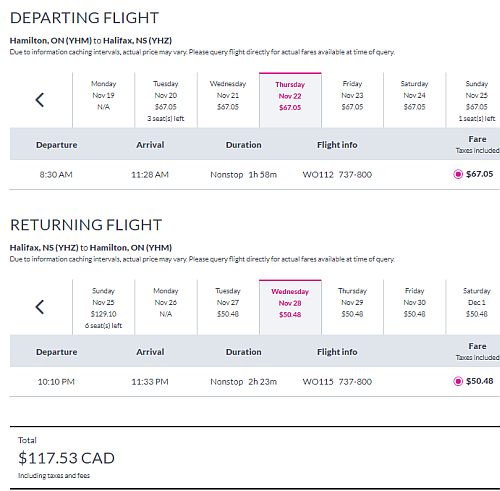**Caption:**

This is a detailed screenshot of the second itinerary on a travel booking page. At the top of the image, the header "Deporting Flight" is prominently displayed. Beneath this, in smaller black text, are the flight details: "Hamilton, ON (YHM) to Halifax, NS (YHZ)." 

Following the flight details, a disclaimer reads: "Due to information caching intervals, actual price may vary. Please query flight directly for actual pairs available at time of query."

Just below the disclaimer, there is a user navigation section featuring a back arrow, followed by a list of dates displaying flight options for every day of the week from Monday through Sunday. For Thursday, November 22, the flight fare is listed at $67.05, and this option is highlighted in pink, indicating it is currently selected.

Below this selection, a gray bar outlines pertinent flight details labeled as "Departure," "Arrival," "Duration," "Flight Info," and "Fare (tax included)." This organized hierarchy provides a clear view of the flight options and the selected fare, ensuring users can easily identify and compare their choices.